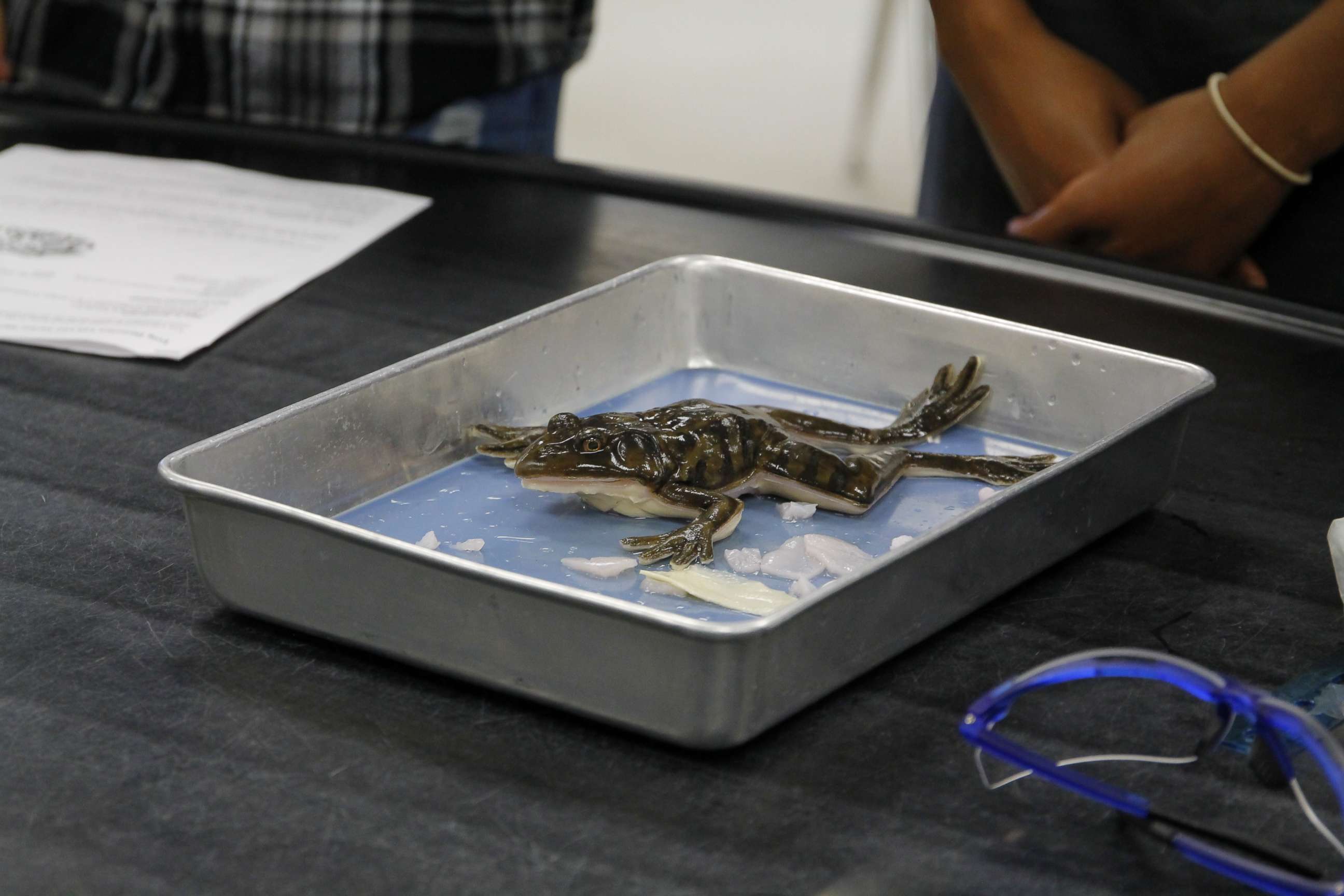In this intriguing photograph, a metallic, gray pen with an almost rectangular shape lies on a dark gray surface. Inside the pen, there is a frog, fully visible and in a lying position. The frog's upper body is predominantly dark green with some black spots, contrasting with its cream-colored lower body. In the background, the partial bodies of two people are discernible, though most of their figures are out of the frame. To the left of the pen, a white paper with text written on it is placed on the surface. Additionally, a pair of eyeglasses is positioned to the right of the pen, adding to the composition's complexity.